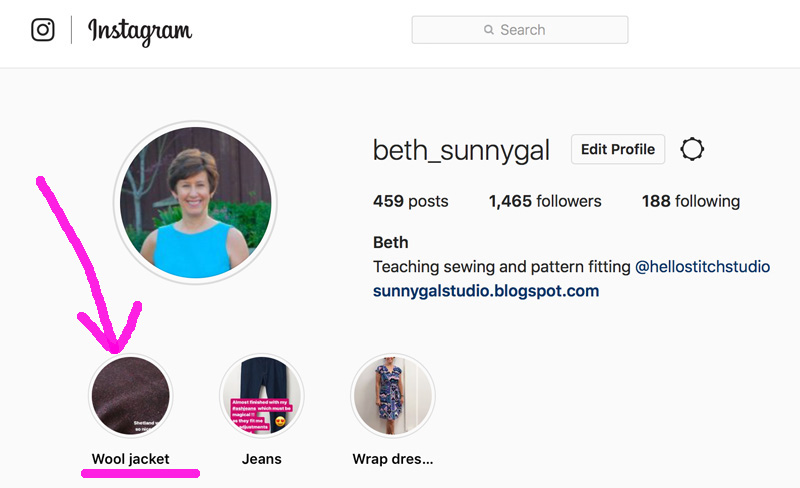The image is a detailed screenshot of an Instagram profile interface. At the top, there’s the Instagram logo and a search bar. Below that, you see the username "Beth_SunnyGal" with a prompt to "edit profile." Beth has 459 posts, 1,465 followers, and is following 188 accounts. Her bio describes her as teaching sewing and pattern fitting at Hello Stitch Studio, and provides a link to her blog, sunnygalstudio.blogspot.com. On the left is a small circular profile picture of Beth, who appears to be smiling in a tank top. Below her bio, there are three smaller circular thumbnail images labeled "Wool Jacket," "Jeans," and "Wrap Dress," with pink arrows pointing towards them. The background of the interface is light gray, and a darker font is used for the text, further enhancing the clarity of the profile details.